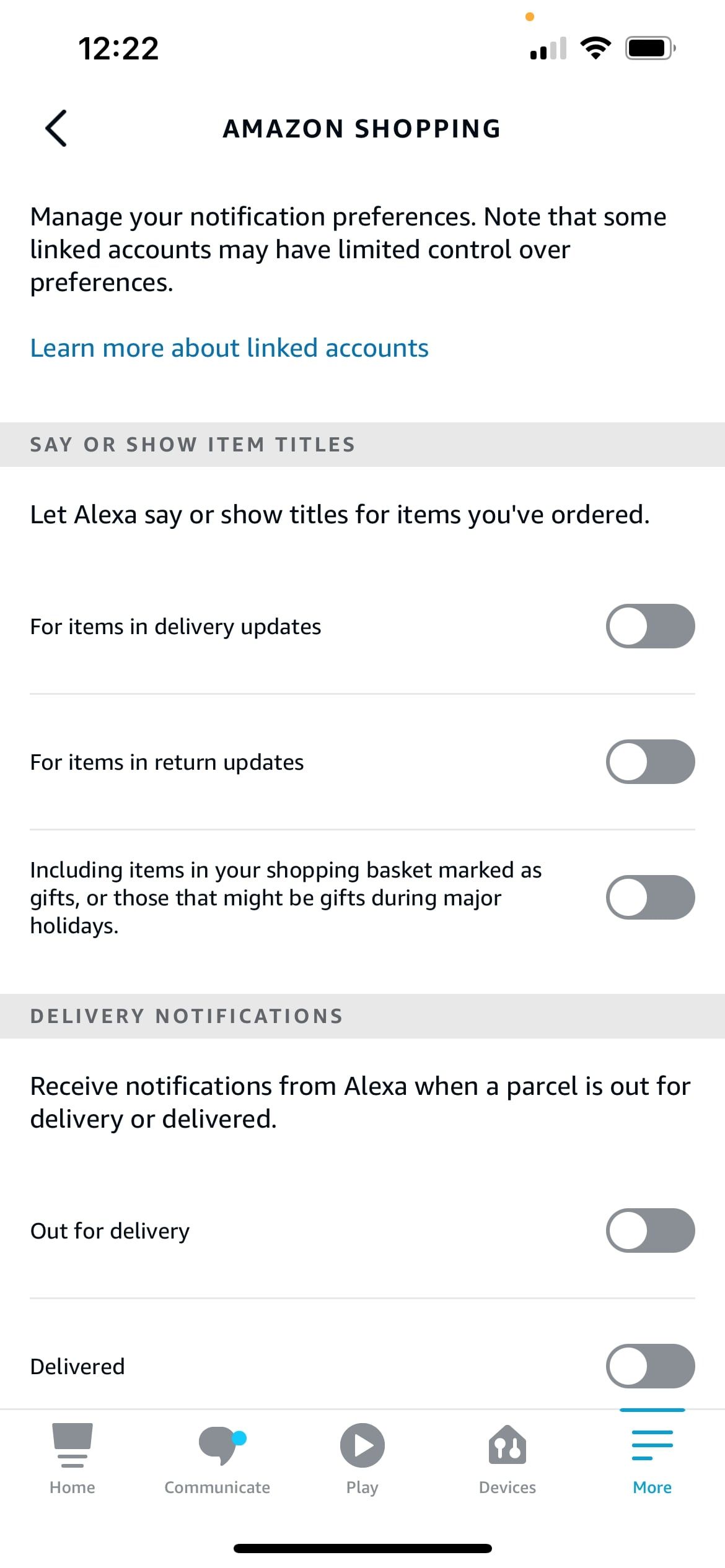The image features a white background with the time displayed as "12:22" at the top. On the left side, there's an arrow labeled "Amazon Shopping." Below, there's a section titled "Manage your notification preferences," with a note stating that some linked accounts may have limited control over preferences. In blue text, there's an option to "Learn more about linked accounts."

A gray rectangle contains the heading "Say or show item titles," followed by a description allowing Alexa to vocalize or display titles for items you've ordered. Several toggles are listed below:

- For items and delivery updates, the toggle is set to "Off."
- For items and return updates, the toggle is set to "Off."
- For items marked as gifts or those that might be gifts during major holidays, the toggle is set to "Off."

Another gray rectangle titled "Delivery Notifications" informs users that they can receive notifications from Alexa when a parcel is out for delivery or has been delivered. Two more toggles are listed here:

- Out for delivery, the toggle is set to "Off."
- Delivered, the toggle is set to "Off."

At the bottom of the image, there's a navigation bar with icons labeled "Home," "Communicate" with a blue dot, "Play," "Devices," and "More" (highlighted in blue). This bar sits above a black footer at the very bottom.